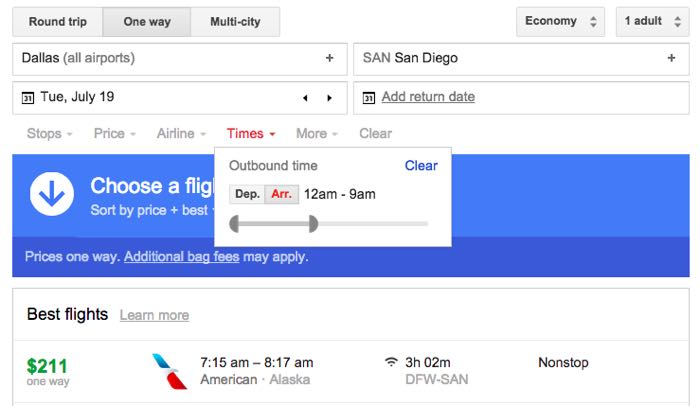The image showcases a detailed flight booking interface. In the upper left-hand corner, there are tabs for selecting the type of trip: "Round Trip," "One-Way," and "Multi-City." To the right of these tabs, there are options to select travel class under the "Economy" tab, and the passenger count indicated as "1 Adult," both featuring up and down arrows for adjustment.

Beneath this row, there are input fields for selecting departure and destination locations. The first input field on the left is set to "Dallas, All Airports," accompanied by a plus button. To the right, the destination input field is set to "San Diego," also featuring a plus sign within the box.

Directly below the destination field is a date selector box showing "Tuesday, July 19th." Adjacent to this is an "Add Return Date" input box for choosing the return flight date. Lower down, a menu bar with options for refining the search further is visible, listing categories such as "Stops," "Price," "Airline," "Times," and "More." There is also a button labeled "Clear" for resetting the search criteria.